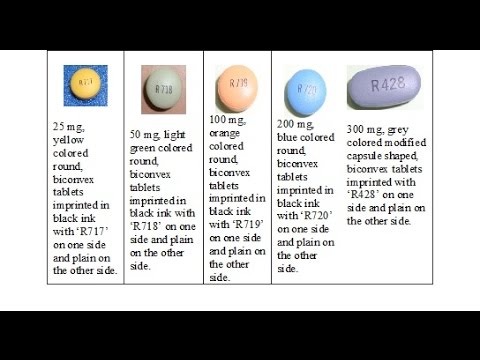This detailed description is focused on an image that appears to be a promotional graphic from an online prescription drug retailer, showcasing five different tablets. The image is framed by a thick black border on the top, bottom, and sides, enclosing a central white background. 

Inside this central rectangle, each tablet is displayed within its own vertical section, separated by thin lines. The tablets vary in size, shape, and color, and include brief descriptions beneath them.

1. On the far left, there is a yellow tablet displayed against a blue background. The yellow tablet features some illegible numbers or letters on its surface.
2. Moving right, the next tablet appears light gray and is set against a beige background.
3. The center tablet has no additional background and sits directly on the white center rectangle. It has a peach or pinkish hue.
4. Next, a sky blue tablet is displayed.
5. On the far right is an oblong, purple tablet. This tablet has a visible imprint reading "R428" and a detailed description below. According to the description, it is a 300-milligram, modified capsule-shaped, biconvex tablet, identified by "R428" on one side and plain on the other.

Overall, the image is a clean and informative graphic likely used to provide visual identification and detail for different prescription tablets available through an online pharmacy.